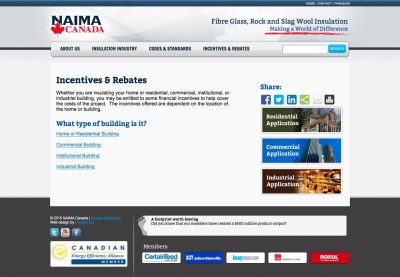**Descriptive Caption:**

This image appears to be an advertisement for a business, likely specializing in insulation products for buildings. At the very top of the advertisement, a thin blue border runs across with some barely visible white text on the right side. Below this border, the main heading reads "NAIM NAIM" in bold blue capital letters. Centered beneath this, the word "Canada" is prominently displayed in red letters, accompanied by a red maple leaf to its left.

To the right of this heading, the phrase "Fiberglass, Rock, and Slag Wool Insulation: Making a World of Difference" is written in blue lettering, accentuated by a red slash underscore for emphasis.

Below these elements, the ad has several interaction points resembling website navigation tabs with labels like "About Us" and "Installation," though the specific text is unclear. A search box is also present adjacent to these tabs. Further down, the text "Incentives and Rebates" stands out in a darker color with additional black text beneath it that is difficult to read.

A blue heading asks, "What type of building is it?" followed by four underlined sections whose details are obscured.

To the right side of the advertisement, the word "Share:" appears with a series of social media icons beneath it, including Facebook, Twitter, Indeed, a general share icon, an email icon, and a print icon.

At the bottom of the image, three thumbnail images of buildings are displayed with white text next to them, though the text is hard to decipher. The bottom-most section features a trademark symbol and the word "Members," followed by five different logos that likely represent partner organizations. Additionally, the "Canadian Energy Efficient Alliance" logo is visible in this section.